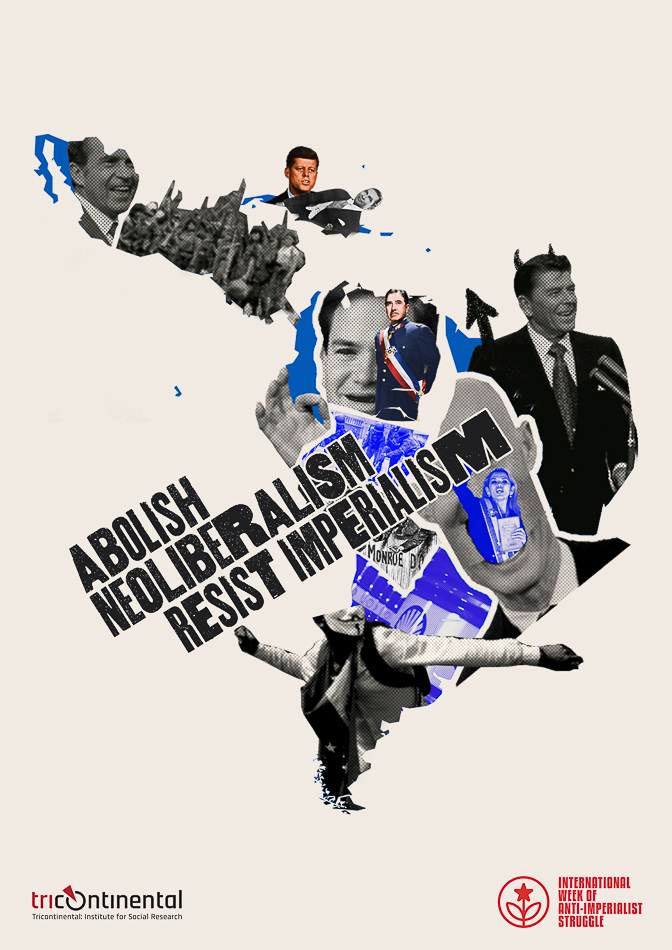This highly political flyer, in a striking black-and-white collage style, carries the bold diagonal message "Abolish Neoliberalism, Resist Imperialism" in large black letters across the center. The upper left corner features a cut-out of Richard Nixon's face, adjacent to another unidentifiable group of people, while just above is an image of John F. Kennedy alongside another indistinct figure. Ronald Reagan appears prominently, embellished with drawn-on horns and a tail, implicating mischief or evil. Below Reagan, a partly obscured figure, possibly Joe Biden, is barely visible. Dominating the lower part of the image is a person wearing a V for Vendetta mask, symbolizing resistance. The poster's base showcases the name "Tricontinental Institute for Social Research" at the bottom, with "International Week of Anti-Imperialist Struggle" prominently in red in the lower right corner. A map in the background hints at a larger narrative connecting historical American leaders to broader geopolitical implications, emphasizing a critique of their policies across Latin America.